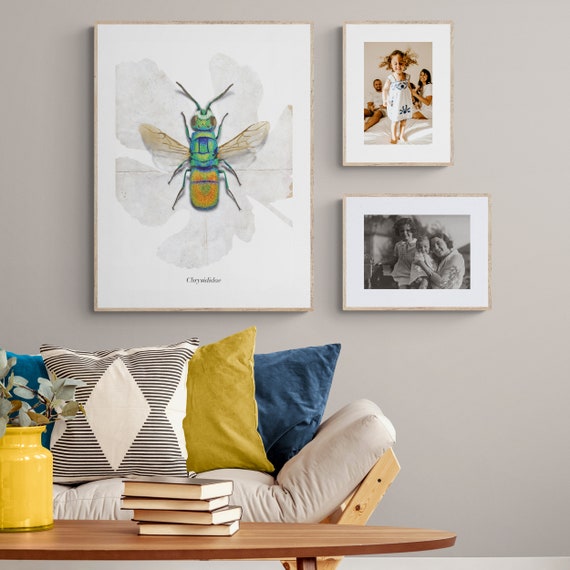In this photograph of an impeccably designed living room, reminiscent of a page from a decorating magazine, there is a silvery pale gray wall adorned with three distinct pieces of artwork. The largest artwork, centrally placed, features a colorful green, orange, and blue insect with translucent wings against a fading silhouette of a flower. At the bottom of this piece, the name of the insect, starting with "CHR," is partially visible. Flanking this on the right are two smaller, white-matted, framed photographs. The upper photograph captures a lively moment of a little girl in a white and blue dress, bouncing joyfully on a bed, her parents seated behind her, smiling. Below this, an older black-and-white photograph depicts a likely earlier time, featuring either the same couple with their baby, or possibly an older family photo of a woman holding a baby with a man standing beside her, set against an outdoor background.

Beneath this gallery wall is a modern beech wood-framed futon-style sofa, adorned with four visually striking throw pillows: two in teal blue, one in cream and black with a diamond pattern, and another in a subdued golden yellow. In front of the sofa, a low, elliptical wooden coffee table holds a collection of objects—a wide-mouthed yellow vase brimming with eucalyptus branches and a neatly stacked quartet of hardback books, their spines facing away from the viewer, showcasing the white edges of their pages. This meticulously curated space fuses contemporary design with warm, personal touches, creating an inviting and aesthetically pleasing living area.